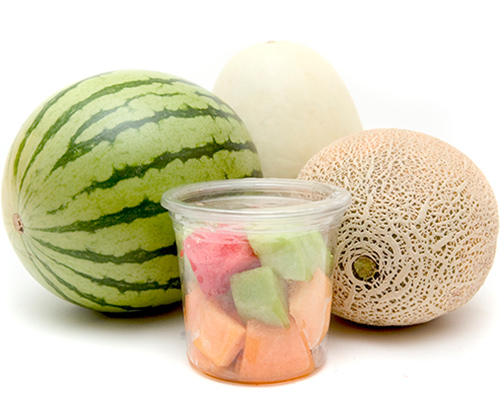This meticulously staged studio photograph showcases a vibrant display of three whole melons—a round, stripy-skinned watermelon, an oblong, smooth and white honeydew, and a netted, speckled brown cantaloupe. In the foreground, a small, clear plastic cup with a lid holds large, colorful cubes of these fruits: the bright red of the watermelon, the minty green of the honeydew, and the peachy orange of the cantaloupe. Set against an all-white background that enhances their vivid hues, the composition is illuminated by an overhead light source, casting subtle shadows beneath the fruits. The professional setting and arrangement highlight the fresh, appealing quality of the melons, making this a visually striking and appetizing image.